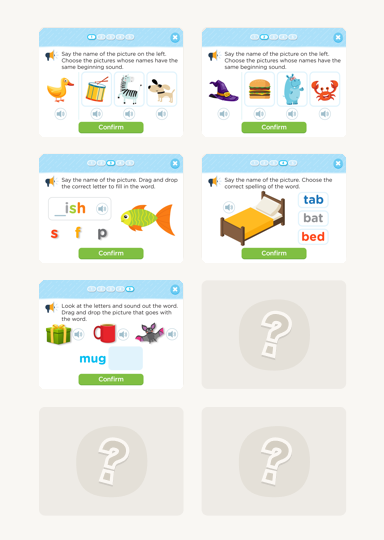This image displays an online product listing for an educational game designed for children, featuring various cartoonish interactive elements. It is organized on a light gray background with no border, structured into two columns each containing four items, forming four rows of two rectangular units.

**Detailed Layout of the Image:**

1. **Unpopulated Tiles:**
   - **Location:** Bottom left of the left column and bottom two of the right column.
   - **Appearance:** These tiles are depicted with a darker gray background featuring a darker gray circle and a question mark icon, indicating they are unpopulated or inactive.

2. **Populated Tiles:**
   - **Number:** Five.
   - **Layout Elements:** Each has a light blue header and border, a white main background, a medium blue circular button with a white X in the upper right corner for closing the tile, and a green button with rounded edges labeled 'Confirm' in white at the bottom center.
   - **Additional Elements:** 
     - **Top Left Corner:** A megaphone icon.
     - **Text Instructions:** Few lines of descriptive text to the right of the megaphone icon.

3. **Row and Column Descriptions:**
   - **Top Left Tile:**
     - **Instructions:** "Say the name of the picture on the left. Choose the picture whose names have the same beginning sound." 
     - **Images:** Duck, Drum, Zebra, Dog.
     - **Interactive Element:** Sound icons beneath each image for auditory feedback.

   - **Top Right Tile:**
     - **Instructions:** Identical to the top left tile.
     - **Images:** Purple witch's hat, Double cheeseburger, Light blue character resembling Barney, Crab.
     - **Interactive Element:** Sound icons beneath each image for auditory feedback.

   - **Second Row Left Tile:**
     - **Instructions:** "Say the name of the picture to the right."
     - **Images:** Fish, with a word prompt showing "_ I-S-H" in various colored letters.
     - **Interactive Element:** Options for letters "S," "F," and "P" in various colors, encouraging the user to select the correct starting letter "F" for "Fish."

   - **Second Row Right Tile:**
     - **Instructions:** "Say the name of the picture to the left."
     - **Images:** Cartoon drawing of a bed.
     - **Interactive Element:** Options for words "Tab," "Bat," and "Bed" in different colors, prompting the user to select the word "Bed."

   - **Third Row Left:**
     - **Instructions:** Contains text that describes an activity involving three images.
     - **Images:** Green present with yellow bows, Red coffee mug, Gray bat.
     - **Interactive Element:** Options beneath images with the word "Mug" in bright light blue, guiding the user to pick the correct image corresponding to the word "Mug."

Overall, the image portrays a structured, interactive educational tool aimed at helping children with word association, phonetics, and vocabulary building through a visually engaging interface.